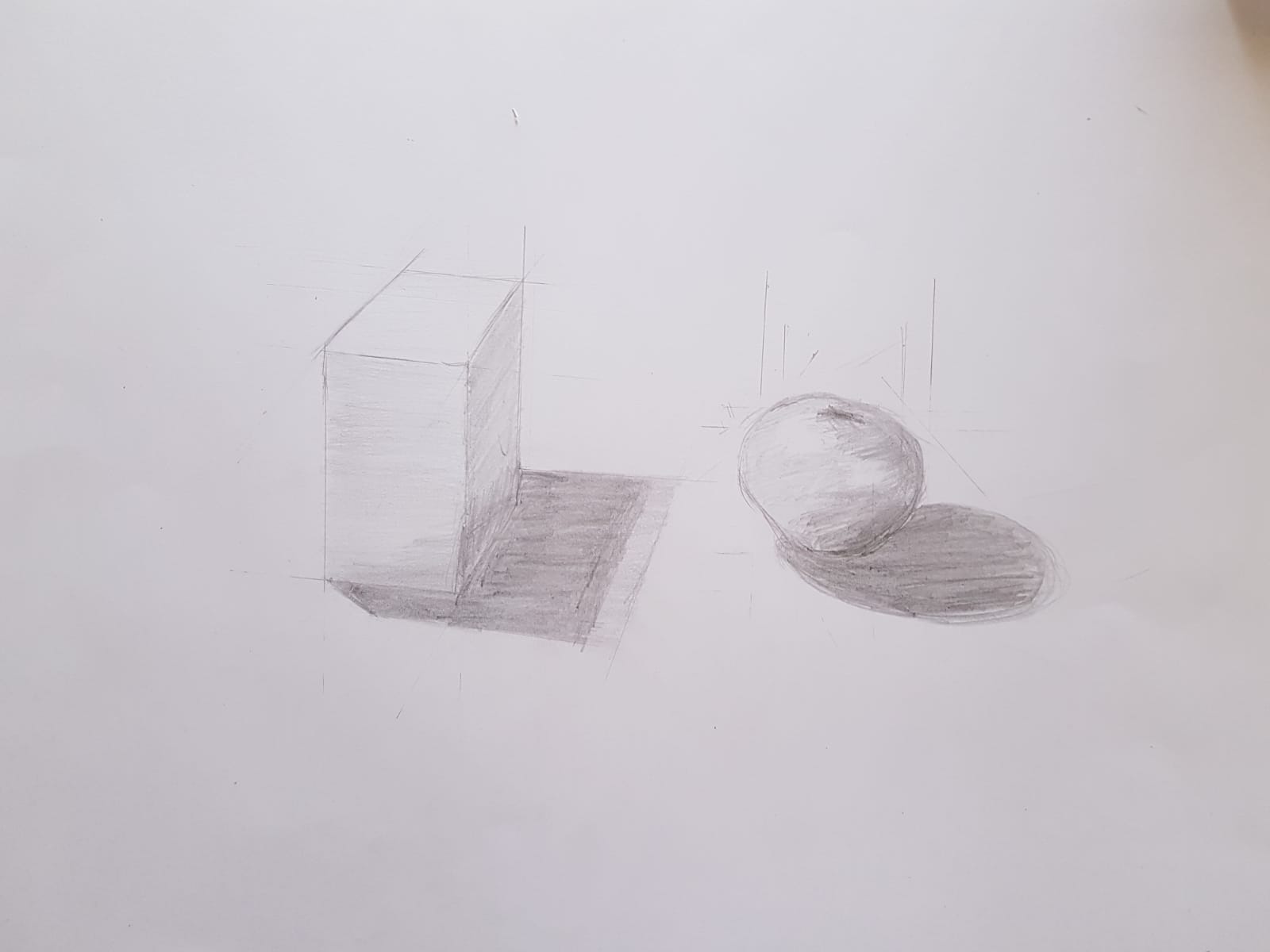This pencil sketch on white drawing paper showcases two primary objects: a sphere and a 3D rectangular cube, both rendered with detailed shading to emphasize their dimensions. On the right side of the drawing, the sphere, resembling a piece of fruit—possibly an orange or a tomato—is depicted with meticulous attention to light and shadow. The left half of the sphere is light gray, transitioning into a darker gray on the right, culminating in a small black circle at the stem area. Fine dark lines texture the sphere, enhancing its rounded and realistic appearance. Adjacent to the sphere, on the left side of the paper, there's a 3D rectangular cube. This shape is white at the top, with structural lines extending to the left and right, reinforcing its three-dimensionality. The left face of the cube is light gray, while the base transitions from light to dark gray, highlighted by a diagonal line that meets a shaded rectangular form in front. This shading gives the cube its 3D effect. Despite one person's interpretation, it appears these forms are not part of a larger scene but are individual studies of shapes and shadows. The artist’s pencil work is evident in the precise delineations and the handling of light and shadow to create depth.